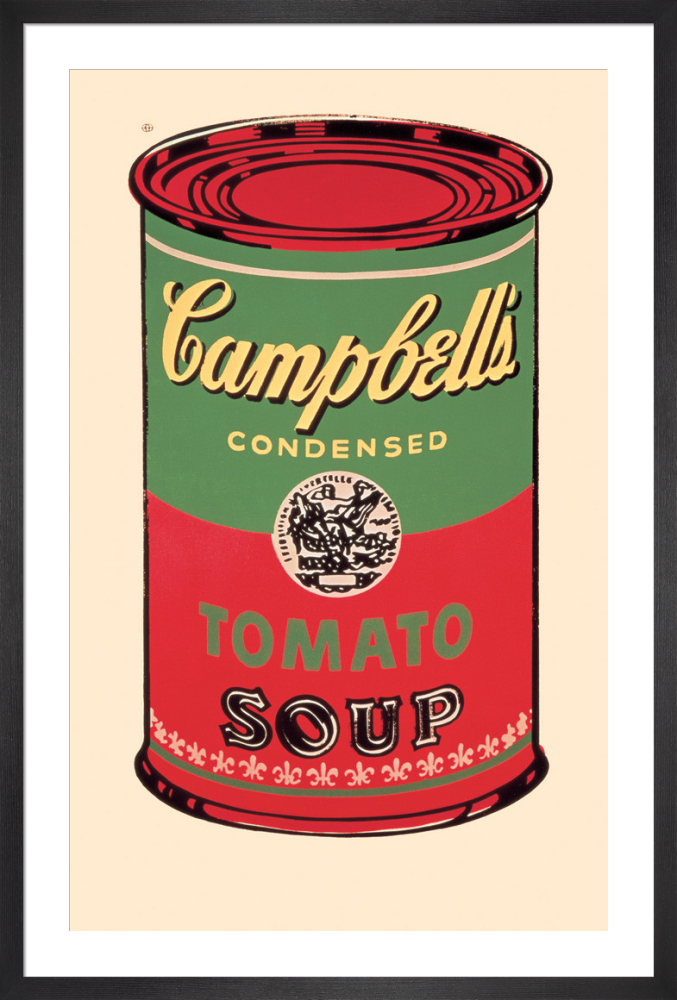This image depicts a stylized, retro drawing of a Campbell's Condensed Tomato Soup can, designed in a vibrant pop art style. The can features a striking color shift: the lid and bottom lip, typically silver, are rendered in bright red. The can itself is framed by a very thin black plastic frame with a white mounting card. The background of the image is a very light salmon color, which adds a nostalgic feel to the overall composition.

In detail, the top half of the can's label is colored green with the word "Campbell's" written in a light yellow color, slightly outlined in black. The word "Condensed" underneath is also in yellow. A black drawing of a statue on a white background serves as a central logo. The bottom half of the label is red, featuring the word "Tomato" in capital green letters and the word "Soup" in a contrasting black and white font. The label is further accentuated by a ring of small white fleur-de-lis along the very bottom, underlined with a thin green ribbon. This combination of colors and elements gives the can an almost festive appearance, seamlessly merging modern pop art aesthetics with vintage design.